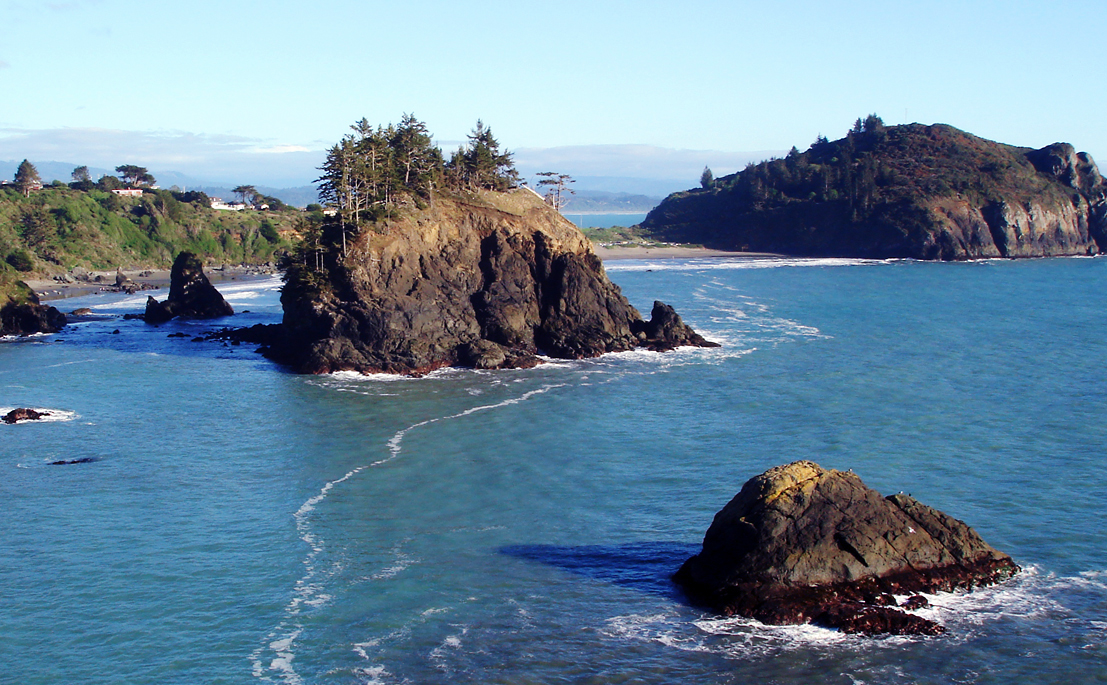This image showcases a picturesque bay, where massive rock formations emerge majestically from a serene, blue body of water. Some of these colossal rocks are so substantial that they support the growth of trees atop them. A peninsula stretches out into the bay, leading to the largest of these rock formations, resembling a mini-mountain. At the base of this imposing rock, cars are parked, suggesting a popular spot that also features a sandy beach. The tranquil area appears to be a favored destination for visitors, likely drawn by the charming beach. On the peninsula itself, several houses perch on a bluff, offering sweeping views of the water and the impressive rock formations in the bay. The calm, beautiful waters add to the tranquil ambiance of this scenic locale.